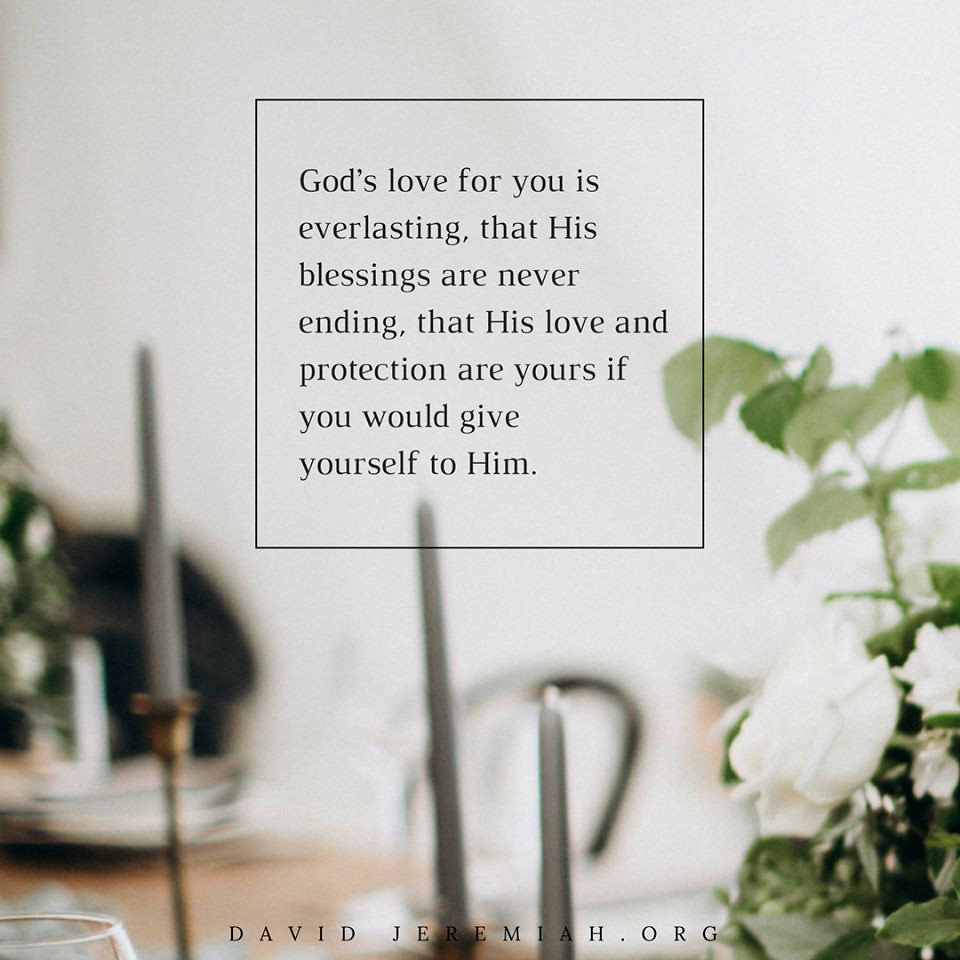The image is a vertical card or meme featuring a background that fades into a blur, with notable elements including a plant, candlesticks, and what appears to be a table adorned with flowers and candles. There are additional elements such as a glass container to the bottom left, and possibly a chair and a stack of bowls or plates in the foreground. Dominantly light blue and white, the image has a rectangular box with dark text placed in the negative space, containing the inspirational message: "God's love for you is everlasting, His blessings are never-ending, and His love and protection are yours, if you would give yourself to Him." At the bottom, in all caps, the website "DavidJeremiah.org" is prominently displayed.